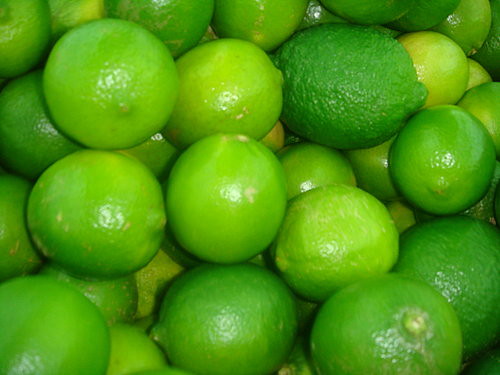This top-down close-up shot showcases a densely packed group of limes, completely filling the frame and extending beyond its edges. The limes are stacked haphazardly, creating a scene where they rest upon one another in an overlapping manner. The image captures various shades of green, from lighter hues to darker tones, highlighting the natural diversity among the limes. While most of the limes are smooth and shiny, reflecting the artificial light source above them, a few stand out due to their bumpier texture, with one particularly bumpy lime noticeable in the upper right corner. All the limes appear fresh, with no signs of rot or disfigurement, and the overall well-lit scene suggests they are contained in a bin or bucket, although the specific container is not visible.